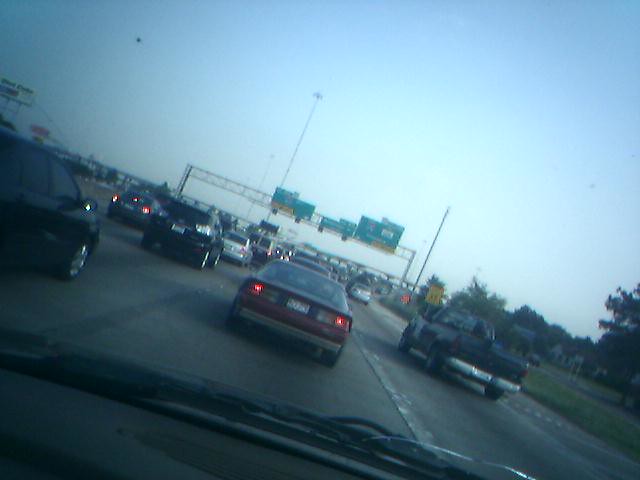This color photograph depicts a bustling traffic scene, likely captured through the windshield of a car. The bottom edge of the image reveals the lower part of the windshield, hinting at the vantage point from inside the vehicle. The entire image is tilted slightly to the right, creating an off-kilter horizon.

In the foreground, there is a dark-colored car with glowing red taillights, indicating a traffic stop or slow movement. To the right of this car is a dark truck, while additional dark-colored cars can be seen on the left side of the scene. 

The bottom right corner features a patch of green grass with trees rising above it, offering a touch of nature amidst the urban setting. The sky overhead is a gradient of light blue, becoming paler towards the center.

In the background, a bridge stretches over the road, adorned with green road signs. However, the signs are too small to decipher their inscriptions. White road lines are visible on the right-hand side, guiding the vehicles along their routes. The overall composition captures the everyday hustle and bustle of a busy roadway, framed by the natural elements of grass and trees against a serene sky.